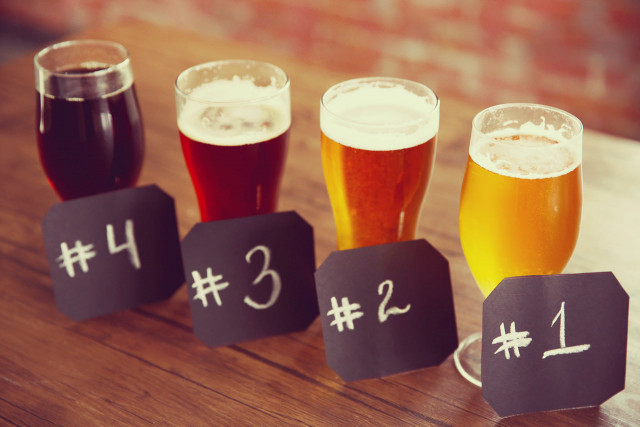In this photograph taken indoors, likely in a pub, we see a rectangular image measuring approximately four inches wide by three inches high. It captures a dark wooden table with subtle black striations and four glasses lined up from the lower right to the upper left. Each glass is labeled with a black signboard featuring white chalk numbers from 1 to 4. 

Starting from the right, glass number 1 contains a light yellow liquid with a frothy white foam on top, suggesting it is a beer. Moving left, glass number 2 holds a darker, golden-orange beer with a thicker foam at the top. Glass number 3 features a dark amber liquid, with a slight head of foam, indicating a deeper brew. Finally, glass number 4, positioned on the far left, contains a deep red, almost brown or black liquid with minimal foam, resembling a robust ale or stout. The blurred background of the image hints at a reddish wood floor, contributing to the cozy pub ambiance.